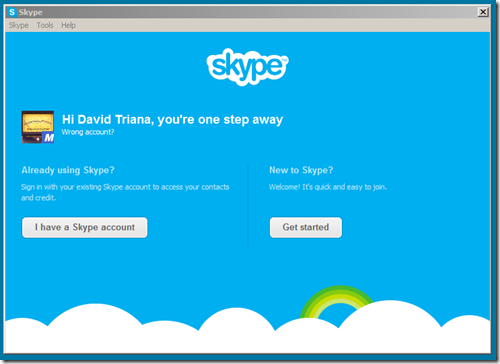Title: Bright and Cheerful Skype Interface

Description: The image showcases the vibrant, user-friendly interface of the Skype application. The dominant color is a bright, cheerful blue that fills the entire background, invoking a sense of energy and positivity. 

In the upper left-hand corner, the iconic Skype logo is prominently displayed. The word "Skype" is written in a smooth, white font reminiscent of a cloud, with a capital "S" standing out distinctly. Just below the logo, there are sections labeled "Tools" and "Help" for easy navigation.

In the top right corner, a small box with an "X" allows users to close the window. Beneath this is a welcome message: "Hi David Triana, you're one step away." Further down, the phrase "Wrong account?" is displayed, possibly offering an option to switch users.

Lower on the screen, there's an illustration resembling a needle and settings icon with the letter "M" on a yellow background, perhaps indicating a tool or a notification.

The main content area invites users to sign in with a pre-existing Skype account to access their contacts and credit. This section includes a white rectangular button that reads "I have a Skype account."

To the right, new users are addressed with a welcoming message: "New to Skype? Welcome, it's quick and easy to use." This is followed by a white rectangular button labeled "Get started."

At the bottom, whimsical elements add to the design's charm: white fluffy clouds and a touch of a green and yellow rainbow-like pathway create a playful, inviting atmosphere, reinforcing Skype's friendly and accessible brand identity.

Overall, the image captures Skype's dedication to providing a bright and user-friendly interface that is easy and enjoyable to navigate.